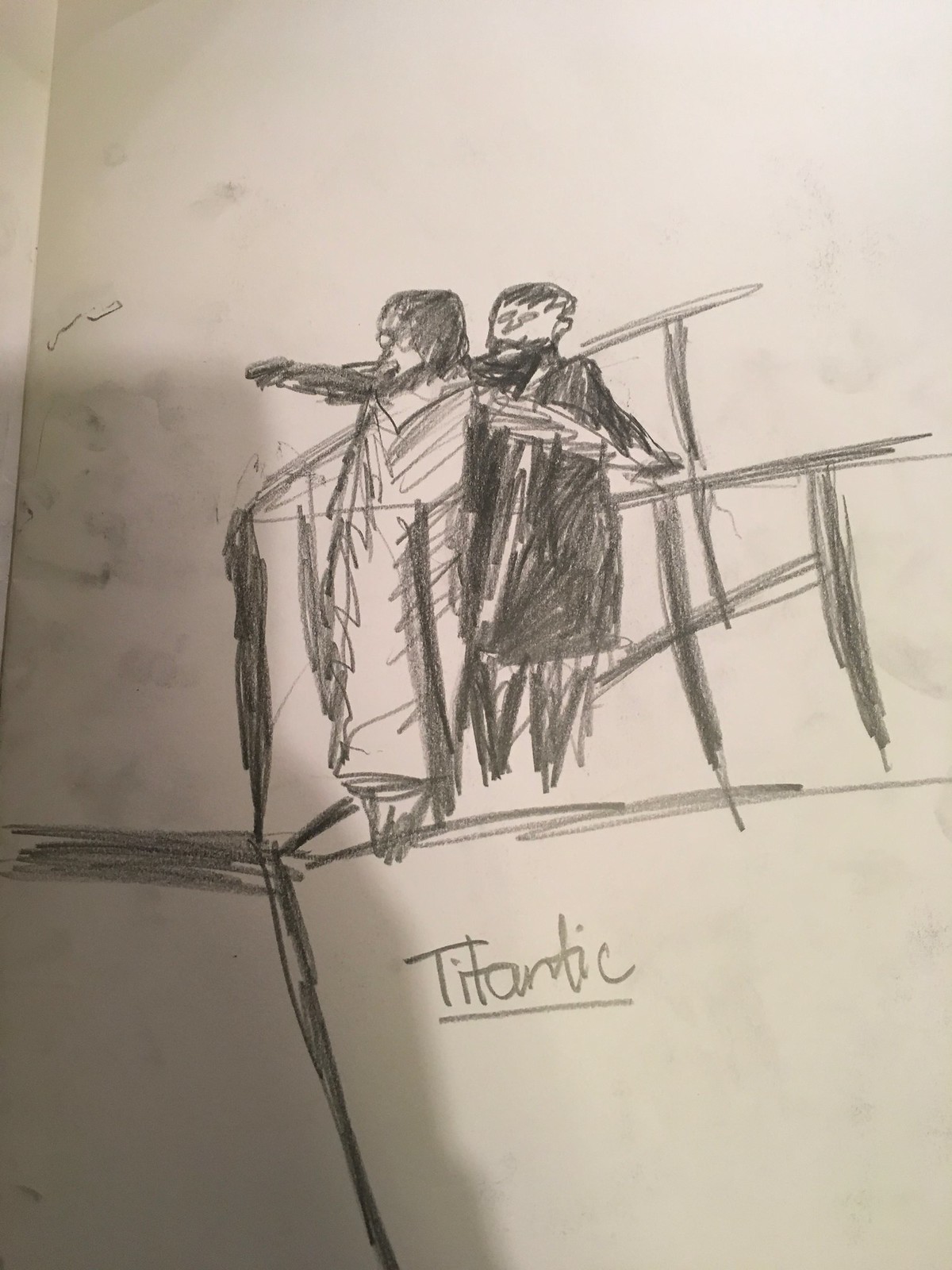This image is a pencil sketch on a blank white piece of paper, featuring a scene reminiscent of a famous moment from the movie "Titanic." The drawing appears to be done with lead, as indicated by the characteristic smudges and strokes. In the illustration, a figure with outstretched arms mimics the iconic pose from the film, where Jack holds Rose at the bow of the ship, giving the impression of flying. The scene includes a basic representation of the ship's railing and part of the vessel, though the details are minimal and the style is rather crude. Both figures of Jack and Rose are also simply rendered, lacking intricate detail. The word "Titanic" is inscribed on the paper, further linking the sketch to the cinematic moment it aims to capture.